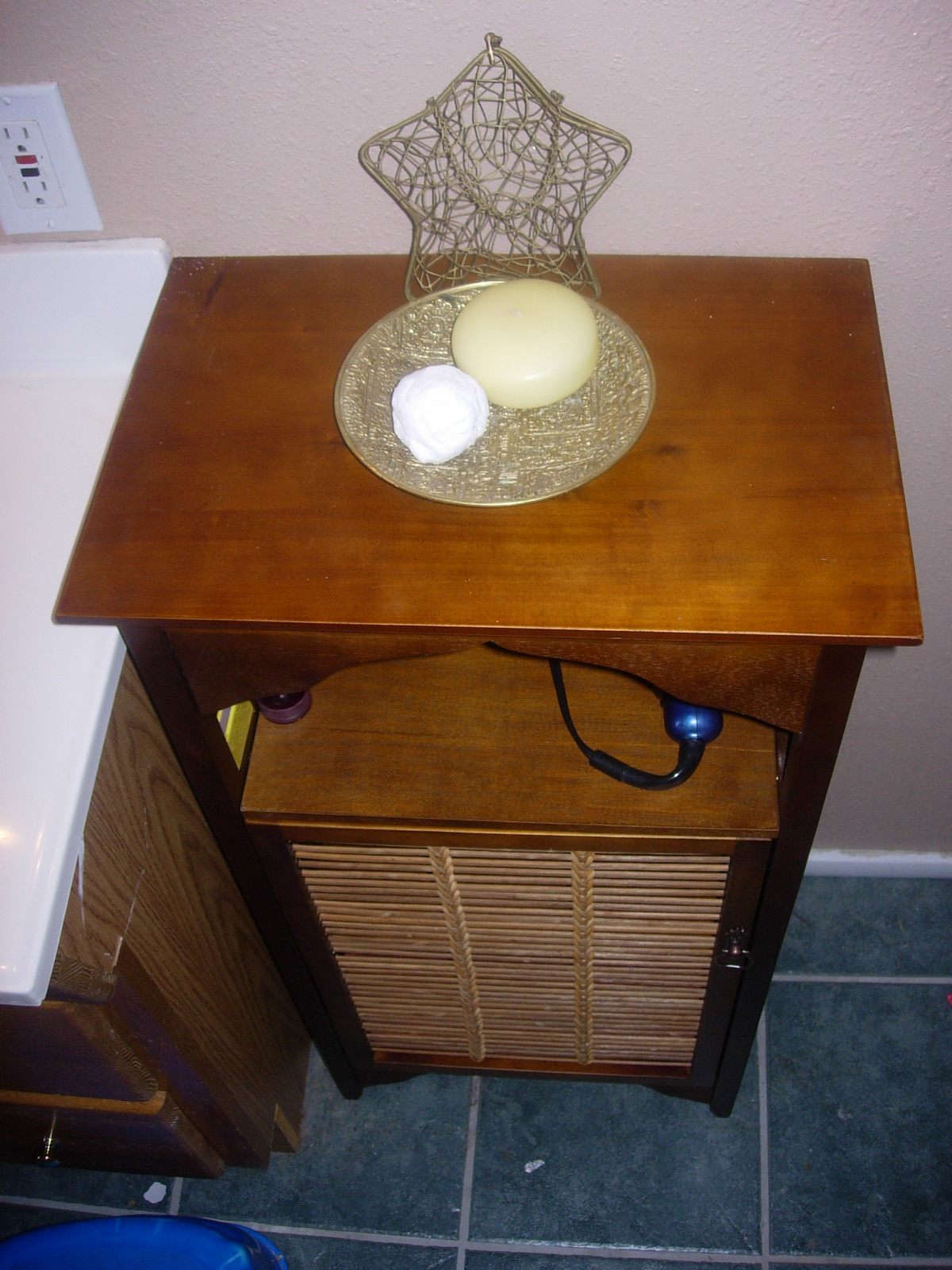A small, intricately crafted wooden side table stands on a medium blue tile floor with gray grout, resting against a wall painted in a soft lilac gray hue. The elegant white woodwork trim subtly accents the scene. Adjacent to the side table, there is a brown wood-grain cabinet, likely made of laminate, which might serve as a bathroom sink due to its shiny white top.

The side table, the focal point of the photograph, is rectangular and unique. On its top, there is a circular silver dish containing two round pieces of soap. Behind the dish is a see-through silver metallic star, adding a touch of whimsy. On the shelf below the tabletop, the handle of a hairdryer or curling iron is visible, suggesting practical storage use. The table's lower section features a door with louvered vents, finished in brown. A small handle on the right indicates the door can be opened to reveal additional storage space inside.